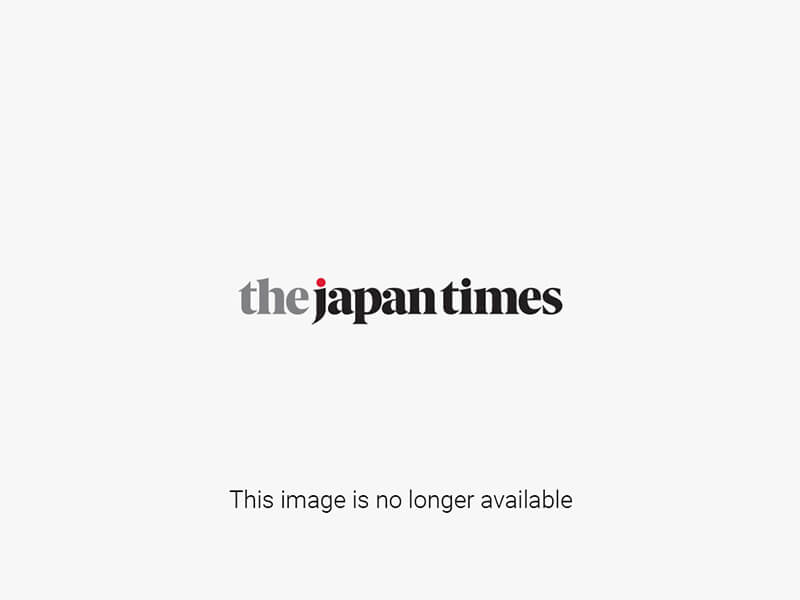In this landscape image, multiple jockeys are seen riding their horses in a thrilling race on a lush green grass field. The jockeys are uniformly dressed in light blue long-sleeved tops coupled with white breeches, some adorned with red accents and polka dots. The leading horse stands out with its dark brownish-red coat, in contrast to the darker-colored horses trailing behind. The scene is set against a backdrop featuring a banner that reads "Longines" twice, as well as partially visible text indicating "Cup GI" and "29 Sunday." Yellow and blue barriers mark the race area, suggesting the horses are nearing the finish line. The overcast sky above adds a dramatic ambiance to the race setting.